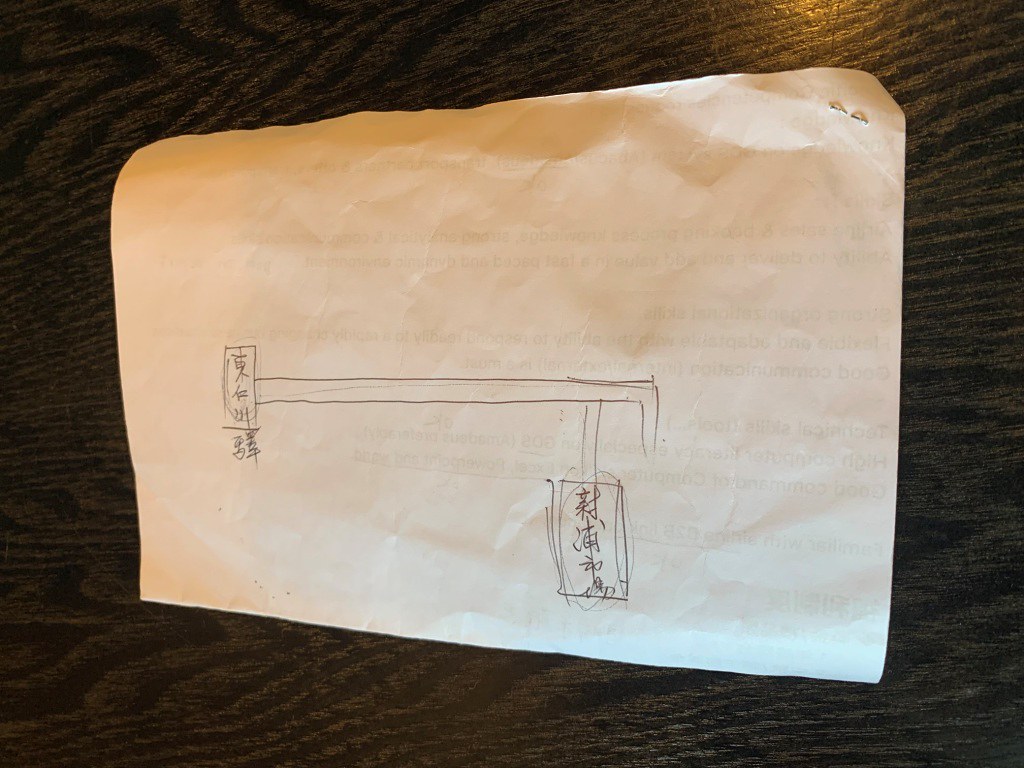This image features a drawing on the back of a stapled sheet of white paper. The front side of the paper contains typed text, but the drawing has been executed on the plain reverse side, likely using a pencil. The drawing comprises a horizontal rectangular shape resembling a snout facing downwards. An arm-like extension emerges from this shape, connecting to a larger rectangular box marked with Asian characters and encircled by a faint, incomplete circle. 

On the left side of the composition, another rectangular box also bears Asian writing, followed by a connecting line and additional Asian characters below it. The artist's intent isn't entirely clear, but the piece appears geometric in nature. The paper, displaying signs of having been flipped, rests on a wooden table, characterized by its dark brown, grainy texture.